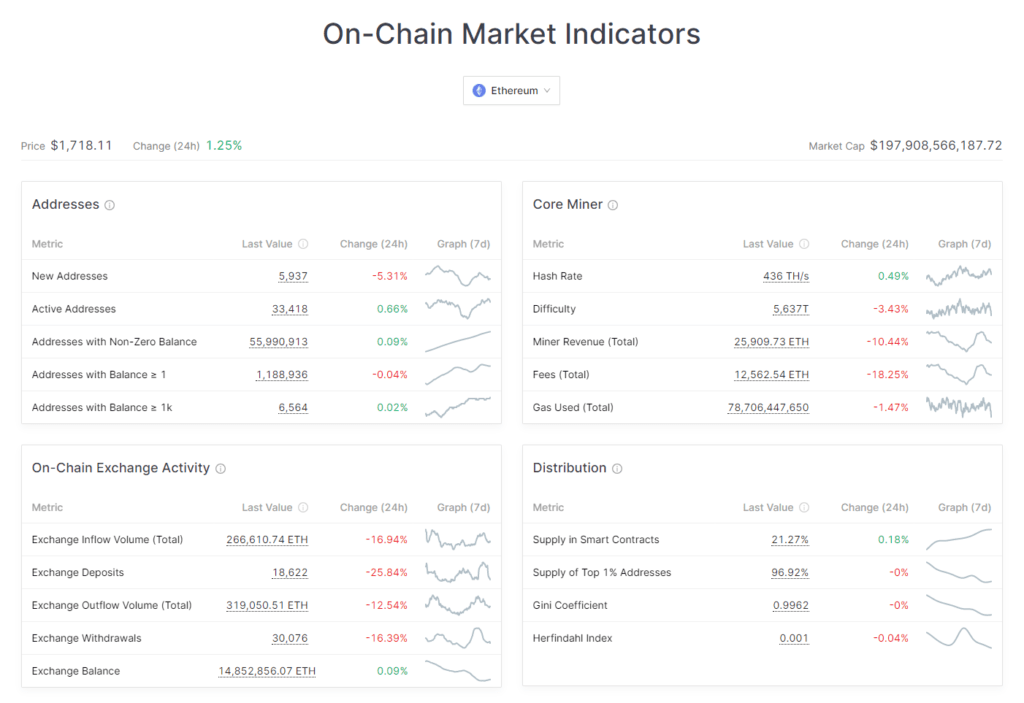This image depicts a detailed screenshot of a cryptocurrency market analysis website, which might be aptly named something like "On-Chain Market Indicators." At the top center of the image, the largest text reads "On-Chain Market Indicators" in black, sans-serif, and title-case font.

Below this heading, centrally positioned, is a rectangle with a gray outline enclosing a blue circle. To its right, the word "Ethereum" appears alongside a drop-down menu, suggesting the ability to select different cryptocurrencies.

On the next row, starting from the left side, the word "Price" is listed with a corresponding value of $1,718.11 next to a dollar sign. Following a small space to the right, the text "Change 24 hours" indicates a percentage change of +1.25%.

Significantly spaced to the right-most side of the image, the term "Market Cap" appears followed by a substantial figure: $197,908,566,187.72. A thin light gray line separates these sections from the contents below.

Further down, the interface is divided into four distinct sections, arranged in a two-by-two grid format. 

- The top-left section is titled "Addresses" and contains rows of detailed information.
- To its right, the top-right section is labeled "Core Miner," displaying rows of data with green and red numbers, as well as small graph icons indicating trends.
- The bottom-left section, under the title "On-Chain Exchange Activity," includes around six rows and four columns, prefaced by information icons.
- Lastly, the bottom-right section, named "Distribution," also features rows of data, each with four labeled columns: Metric, Last Value, Change, and 7-Day Graph.

Each section compiles various metrics related to its title, providing a comprehensive overview of cryptocurrency market indicators.